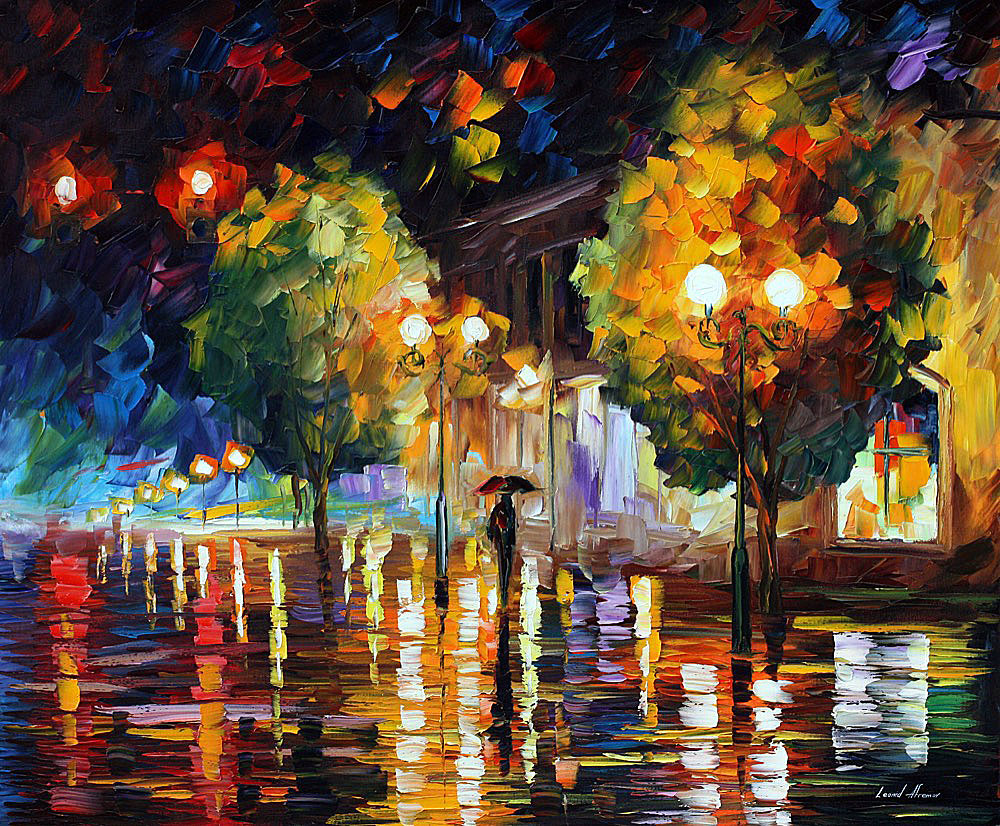This painting captures a vivid and rainy nighttime scene in an outdoor urban setting. A solitary person walks down a wet city street under an umbrella, surrounded by a series of glowing streetlights. The streetlights, each having two glowing orbs, stretch from the top right to the bottom left corner of the image, creating a well-lit pathway. Trees with lush, green foliage frame both sides of the street and are scattered throughout the scene, their leaves displaying a spectrum of colors from lighter greens to autumnal yellows, and deeper oranges and reds under the artificial light. The wet pavement reflects the vibrant colors of red, orange, purple, and white, likely mirroring the illuminated storefront windows to the right. In the backdrop, a brown building with large windows and more trees adds depth to the composition. The painting's style is uniquely blurry yet vivid, enhancing the reflective wetness of the street and the misty ambiance of rain. In the bottom right corner, the painter's signature, cursively inscribed with what appears to be "Leonard H." or "Leonard Homer," provides a personal touch to this atmospheric urban nightscape.